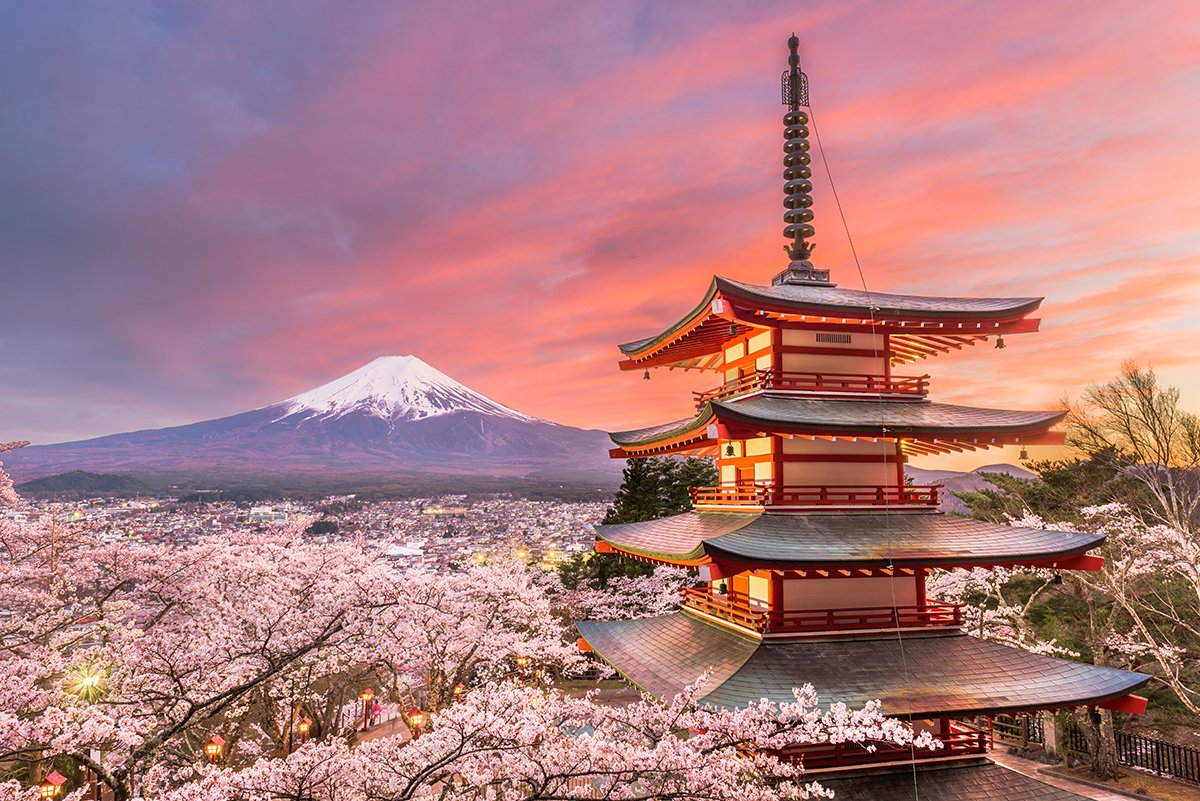This professional photo captures a picturesque scene of Japan during the evening, featuring a traditional four-tiered Japanese building, reminiscent of a Shinto shrine or pagoda. The structure is prominently colored in red and white, with gray or black tiled roofs gracefully separating each tier. A distinctive tower rises from the top, anchored by a cord reaching down to the ground. In the foreground, sakura cherry trees in full bloom display their vibrant pink leaves, accompanied by other lush green trees, creating a vivid natural frame. The background reveals a serene landscape bathed in the warm, multi-hued glow of a sunset, casting blues, pinks, and yellows across the sky. Dominating the horizon is the majestic Mount Fuji, its snow-capped peak standing tall and pristine. Below the mountain, an out-of-focus town subtly blends into the scenery, adding depth without drawing attention away from the main elements of the image.